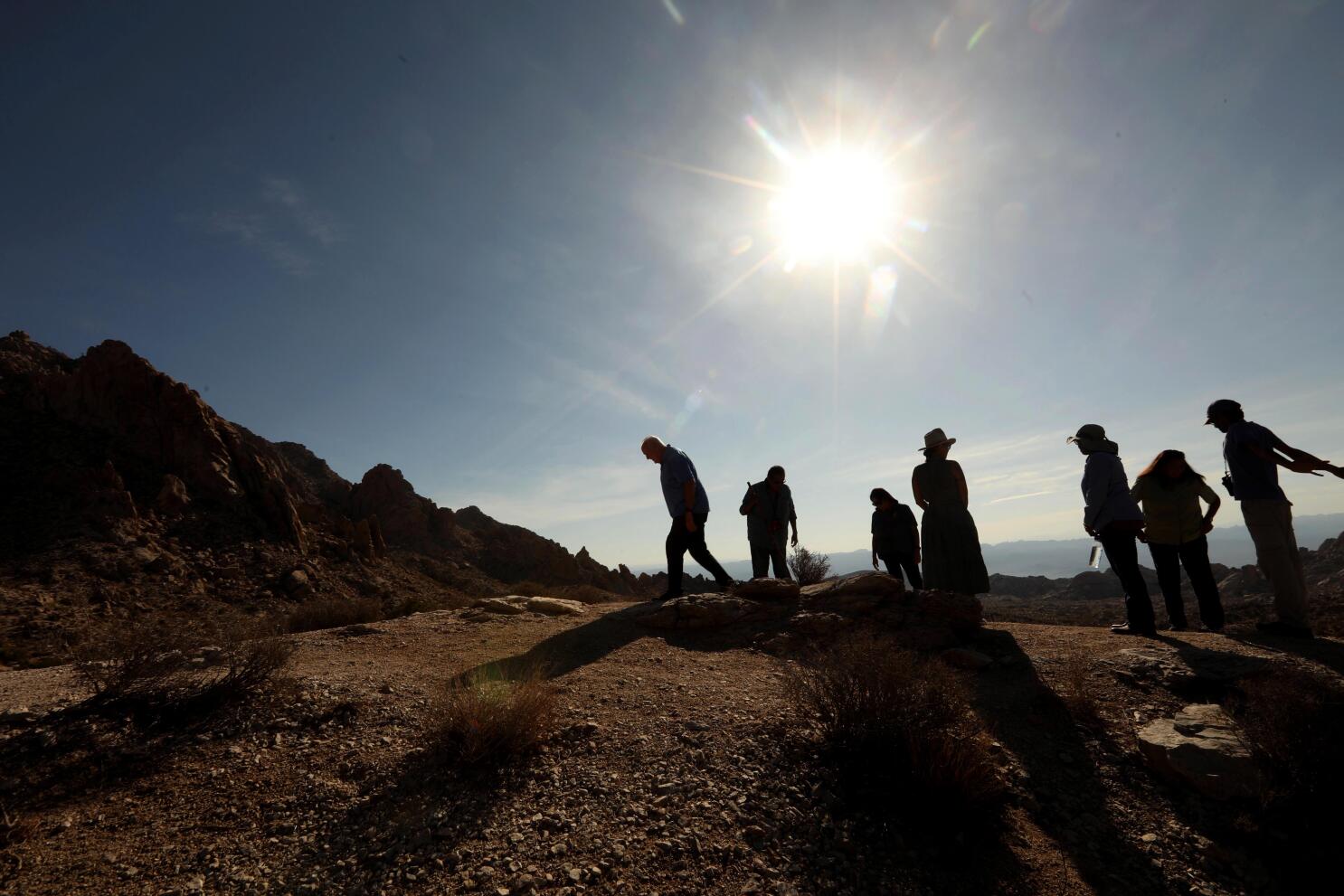This digital photograph captures the striking silhouettes of a group of people standing on a barren, small dirt hill, perfectly framed against a backdrop of a brilliant, high sun and a clear, dull blue sky with minimal cloud coverage. The sun's intense white-yellow light renders the people as dark figures, masking any individual details and creating a powerful contrast in the scene. To the left, a rocky, brown mountain range devoid of vegetation adds to the stark, rugged landscape. The ground itself mirrors the brown tones of the mountains, reinforcing the arid, desolate environment. Despite the lack of detail in the silhouetted figures, the image conveys a sense of camaraderie and adventure, as it appears the group has either hiked or driven to this elevated vantage point to take in the expansive view.